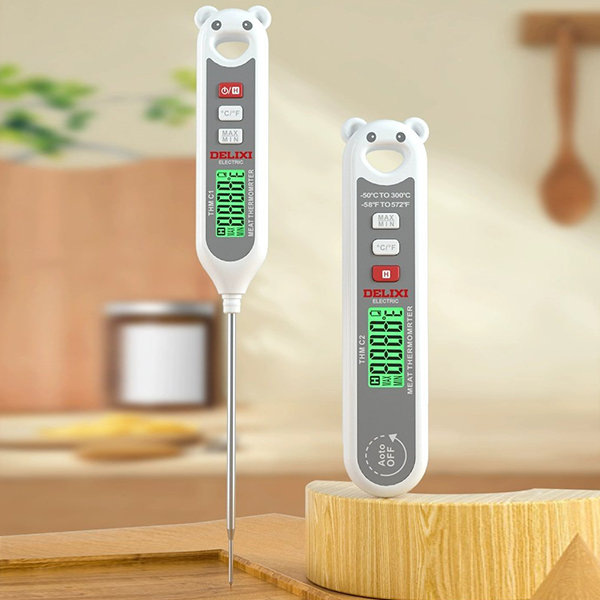In the foreground of the image, there are two digital thermometers designed to resemble teddy bears, characterized by their round ears, circular eyes, and an open-mouth cutout at the top. The thermometers have a white plastic body with a central dark gray panel. Each thermometer features three buttons: one red and two white. The central red button is designated for power, while the two white buttons are likely used for setting Celsius or Fahrenheit and min-max functions. The LCD screens are green and black, displaying various readings. Below the buttons, the brand "Delixi Electronics" is clearly printed.

The thermometer on the right has text indicating "A-O-T-O OFF" along with an arrow and the label "Meat Thermometer," suggesting this one is designed specifically for culinary use. Both devices are equipped with a silver metallic probe extending from the bottom, ideal for precise temperature measurements.

The background of the image is blurred, but hints of a kitchen setting can be discerned. Visible elements include a computer or table, a wall adorned with leaves, and a white hanging object. On a brown surface, there’s a wooden spoon hanging, adding to the ambient kitchen aesthetic. The overall scene is likely taken in a well-used kitchen space, providing a practical and homely backdrop for the thermometers.